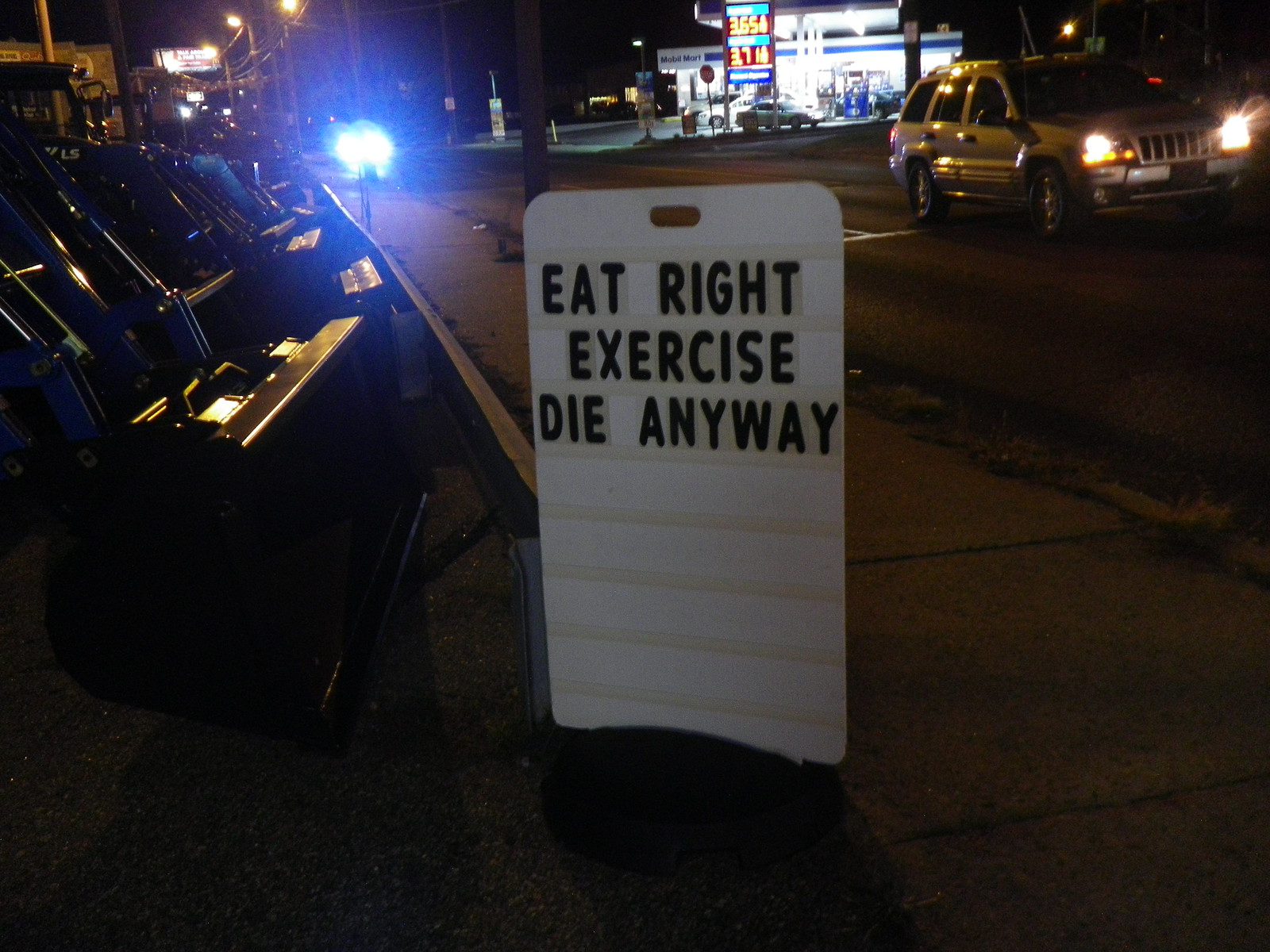In the quiet, dark stillness of a late-night street, a whimsical sign on a sidewalk captures attention with the stark humor of its message: "eat right, exercise, die anyway." The sign, white with black letters arranged in three rows, stands near the edge of the road where a silver vehicle approaches, its headlights cutting through the night. The scene is dimly lit by overhead streetlights, casting a pale glow on the concrete sidewalk divided into multiple squares. Across the street, a brightly lit mobile mart gas station offers a contrasting burst of illumination, advertising unleaded gas at $3.65 per gallon. Additional lights and machinery, possibly arcade machines, stand by, adding to the scene's mysterious ambiance. In the background, electrical wires crisscross the sky, and a distant billboard remains too small to decipher. The overall quietude punctuated by parked cars and the occasional vehicle highlights the eerie charm of this nocturnal urban tableau.